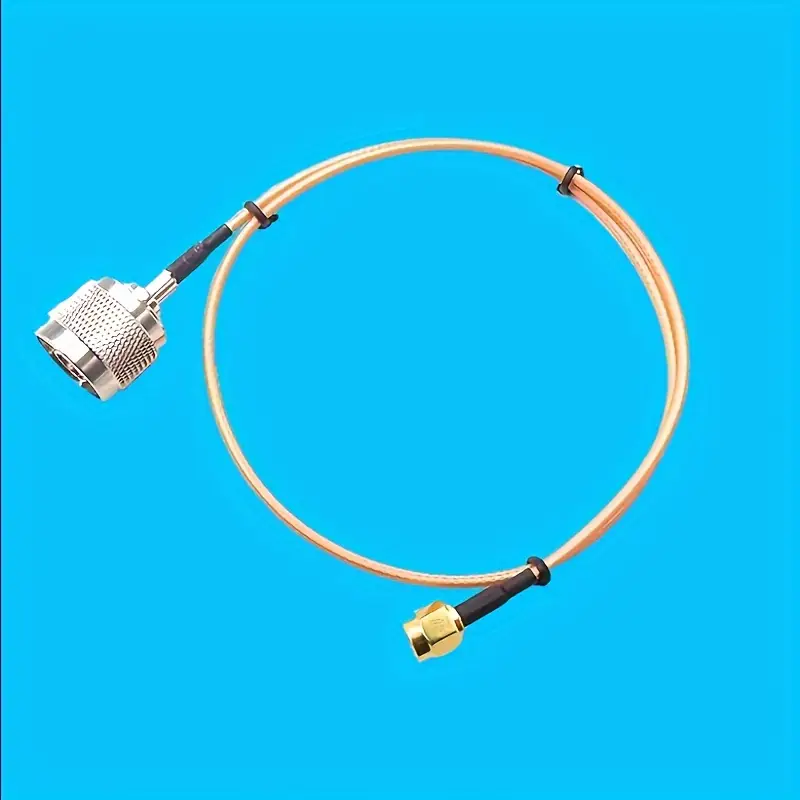In the image, a coaxial cable is coiled into a circular form and secured with three zip ties against a light cyan blue background. The cable has a metallic copper coloration and appears to be about three feet long. Both ends of the cable are visible and distinct. On the left, the larger end features a shiny, textured chrome metal nozzle typically used for hand-tightening, with black tape wrapped around the base where it meets the cord. This end resembles a faucet adapter. To the right, the much smaller end is gold-colored, with a hexagonal bolt, also attached to the cord with black tape. The image is well-lit with flat, even lighting, suggesting it might be a stock photo.